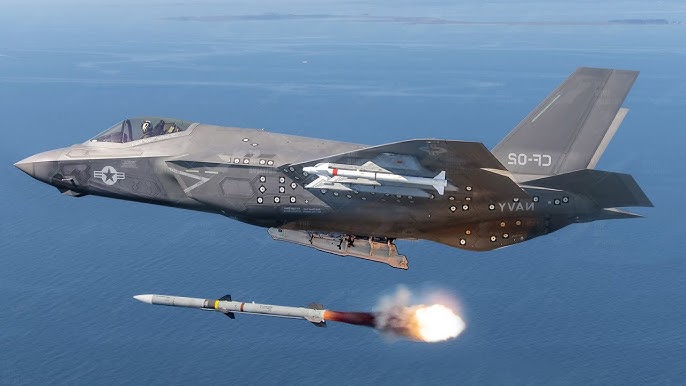In this striking color photograph, a gray US Navy fighter jet is captured in mid-flight over a vast expanse of deep blue ocean. The sleek aircraft, identifiable by its Navy insignia and the white star logo near the cockpit, is shown from the side, with its nose pointing left and its tail on the right. The jet displays markings on its angled tail wing, including the reversed text "CF-02" and "NAVY." Through the glass canopy, the pilot is visible donning a white helmet. Mounted under its wings, various missiles are clearly seen, highlighting its armament.

The focal point of the image is the dramatic launch of a white missile from an open hatch beneath the jet. The missile, adorned with a white tip and colored bands, is depicted with flames and smoke shooting out from its rear, indicating it has just been fired. This powerful scene, set against the serene and uninterrupted backdrop of the blue ocean, captures both the precision and the formidable capability of modern military aviation.